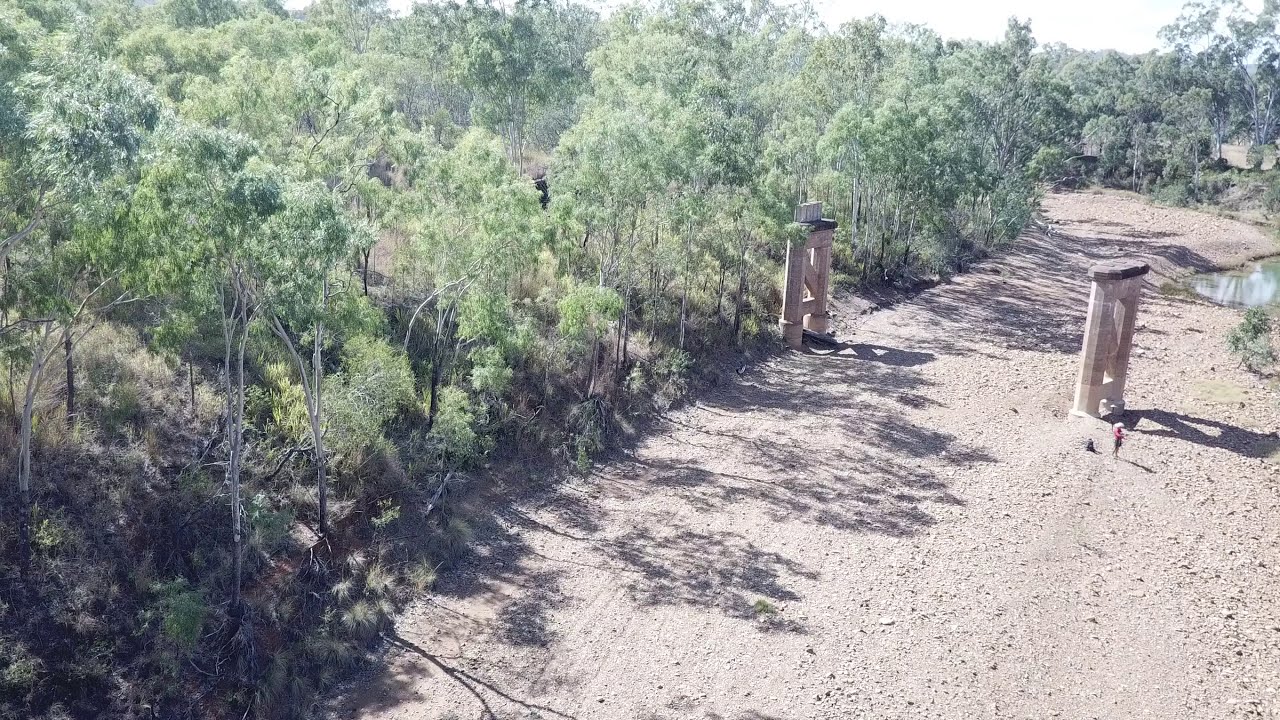The image depicts an outdoor scene with a dried-up riverbed dominated by tan gravel and rocks, bordered on the left by lush greenery. The left side showcases a hill densely populated with light-green trees, their thin trunks and branches catching the light. In the center and slightly to the right of the image, stand two large, tan concrete pillars. These pillars appear to be the remnants of a bridge or overpass, with no visible bridge structure remaining. A woman, dressed in a dark-colored skirt and a red top, stands at the base of the right-most pillar. She is small and indistinct due to the distance. To the far right of the image is a patch of murky green water, suggesting the previous presence of a river, now mostly dried up. The scene captures a moment of desolation and natural reclamation under ample daylight.